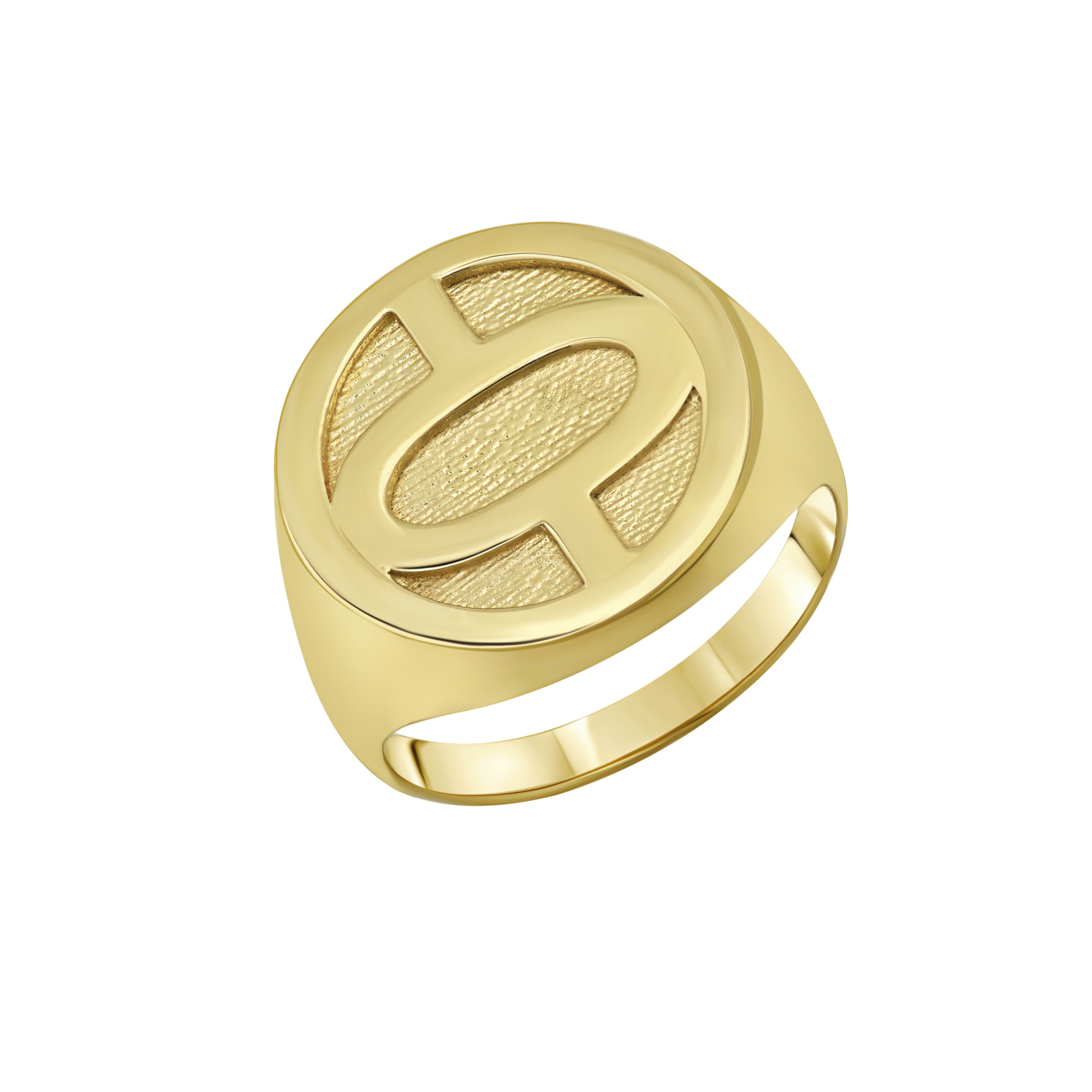This is a color photograph of a signet ring rendered in a vibrant gold or champagne color, giving it more of a satin sheen rather than a shiny appearance. The ring, viewed from a slightly elevated angle that shows both the band and the face, is simplicity incarnate with a solid, plain design. The face of the ring features a peculiar symbol set within an oval, which is further detailed by two lines extending from the top and bottom edges, creating an almost cross-like effect. The surface of the symbol matches the ring's texture, which has a slight beveling. The background behind the ring is a rough, almost brick-like surface, adding a stark contrast to the ring's smooth, polished finish.